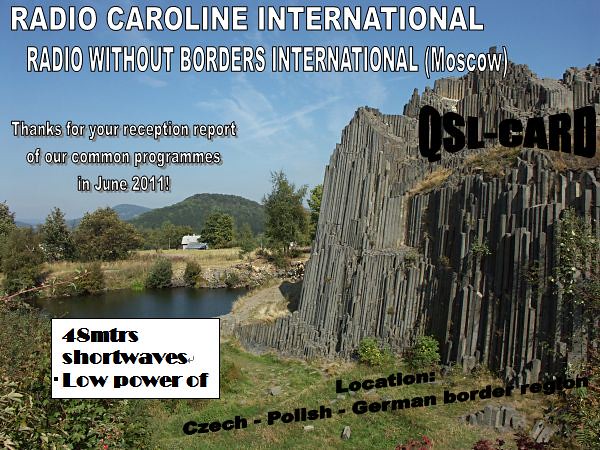This advertisement features a wide rectangular outdoor photograph showcasing a stunning natural landscape. Dominating the right side is a massive, gray rock formation with rugged, ridged edges. To the left of the cliff, lush green hills dotted with trees and patches of grass gently roll into the distance. In the middle of the scene, a small, still pond reflects the serene surroundings. The backdrop features a clear blue sky adorned with white clouds, enhancing the beauty of the entire setting. A house is subtly nestled beneath the mountains in the background. 

Overlaying this picturesque landscape, white text at the top left reads: "Radio Caroline International, Radio Without Borders International (Moscow)." Below it, in gratitude for listener engagement, the text continues: "Thanks for your reception report of our common programs in June 2011!" At the bottom of the image, underneath the pond, a white box with black text details: "48 MTRS shortwave low power OF," highlighting its broadcasting reach. Additionally, "Location: Czech-Polish-German border region," is noted, pinpointing the geographical focus of the advertisement. Adding a touch of intrigue, the word "Oslo" (spelled "O-S-L-C-E-R-D") appears in the top right corner.